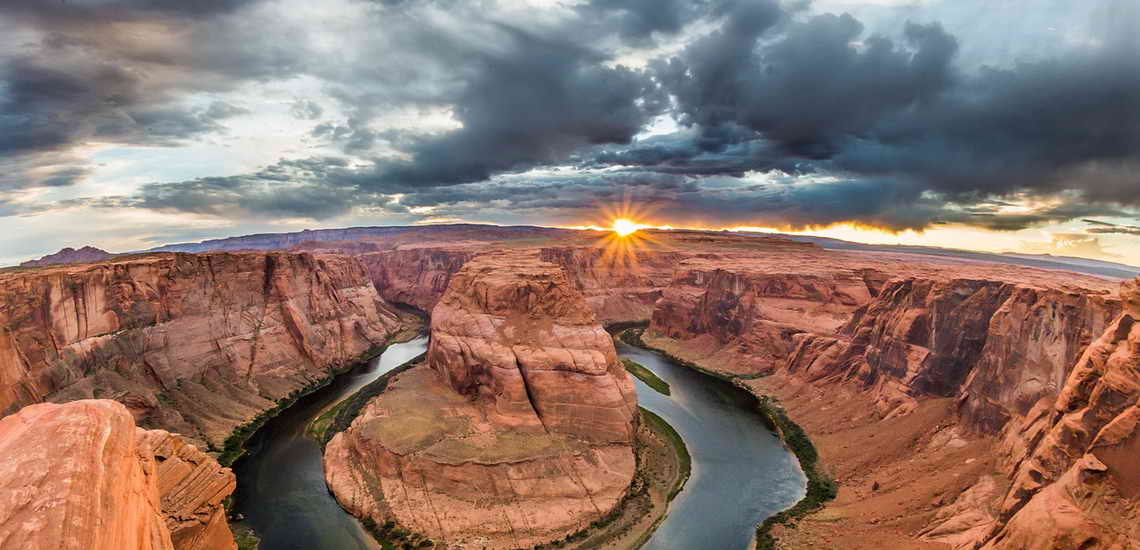The image captures a highly detailed, photorealistic yet stylized panoramic view of a canyon reminiscent of the Grand Canyon. The deep, U-shaped canyon, sculpted over millennia, has striking striations in its steep, orangish-brick-red cliffs, suggesting southwestern terrain. Centrally, a majestic rock formation stands encircled by a dark blue river or lake, with patches of grass and vegetation dotting the banks. The sky above is dramatic, with a small, glowing sun peeking just above the horizon during sunset, painting the horizon bright yellow and fading to purples while darker clouds loom overhead, possibly hinting at impending rain. The overall impression is one of vast, rugged beauty, viewed as if from a high vantage point on another cliff, encapsulating the timeless grandeur and complex geology of this awe-inspiring landscape.